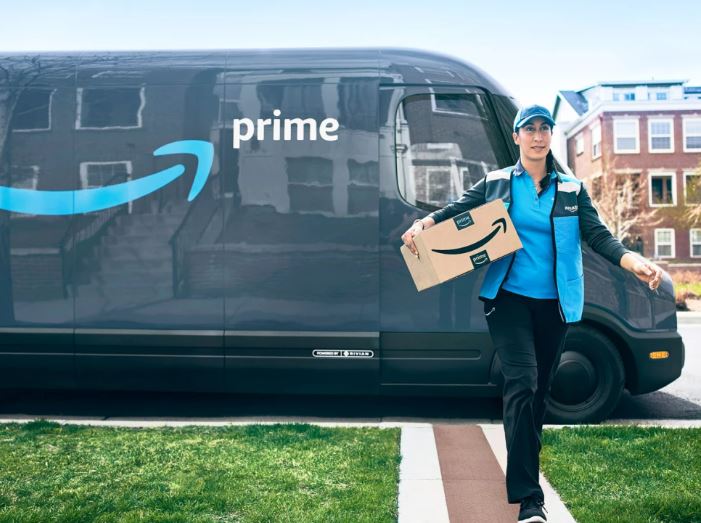In this vibrant photograph, a dark bluish-gray sprinter van with a large reflective side panel occupies the background. The reflective panel showcases a walk-up apartment building constructed of brick, with prominent concrete steps leading to its entrance. The left facade of the building appears darker, while the right is lighter. Decorated on the van’s side is a large, blue arcing arrow pointing to the white text that reads "Prime".

In the foreground and to the right of the van, stands a woman dressed in black pants and a blue shirt layered with a jacket that transitions from blue at the bottom to dark blue at the top. She also dons a blue hat. She walks towards the camera along a small pathway marked by a red stripe down its center and bordered by white. The woman’s left arm is extended and she firmly clasps a light brown box against her waist with her right arm. The box features a black arcing arrow and is sealed with black tape adorned with white text that spells "prime," accompanied by a smaller white arcing arrow.

Behind the van on the right, a four-story house looms in the background, its bottom three stories made of brick while the top floor features white siding and a black, angled roof. The sky overhead is a serene pale blue, providing a tranquil backdrop to this bustling urban scene.